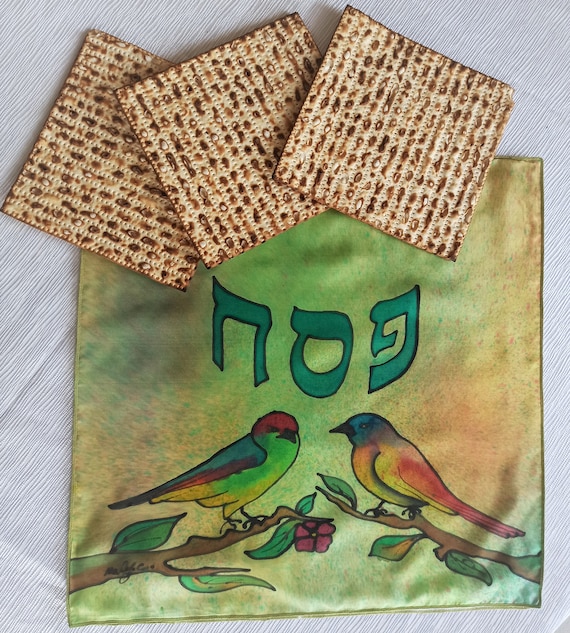This detailed photo captures a Passover matzah cover with a white background. Three square pieces of matzah, tan with toasted brown elements, are arranged with their edges overlapping slightly. The cloth cover beneath the matzah features a central word in Hebrew, composed of three thick green letters outlined in black, resembling "NOG." Below this text, two multicolored birds—one with a greenish body and red head, and the other with a yellowish body and blue head—are depicted facing each other. They sit on separate brown branches adorned with a single pink flower. An artist's name is partially visible on the cloth cover. The intricate details of the fabric design, including the vivid colors of the birds and the delicate floral accents, create a striking and culturally rich image.